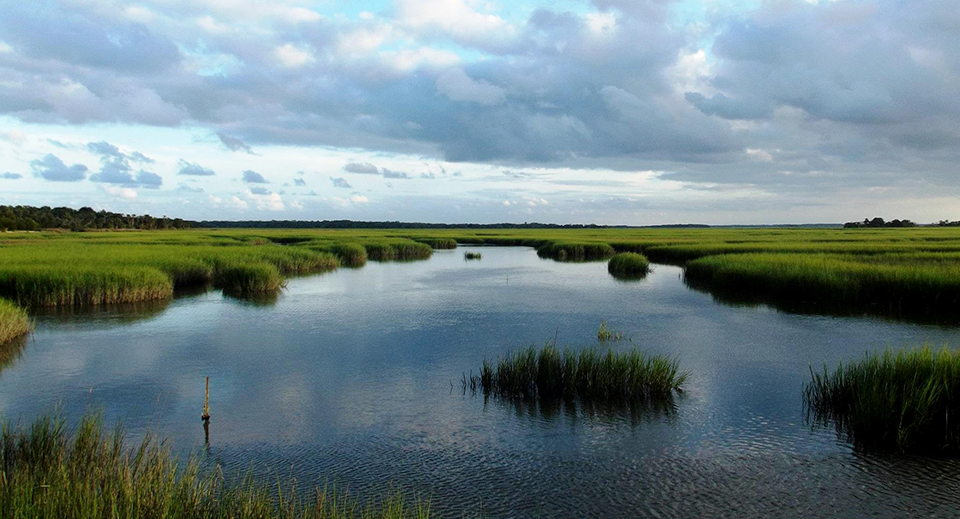The photograph captures a serene daytime landscape dominated by a small lake. The sky above is heavily clouded, casting a shadow over the scene and giving the water a dark blue hue. Occasionally, patches of blue sky peek through the dense clouds, hinting at the sun hidden behind them. Surrounding the lake are various patches of vibrant green grass, with notable brightness on the left side, likely touched by sunlight breaking through the clouds. The right side of the image features darker grass areas, engulfed in more shadow. In the foreground, the shallow water is interrupted by rushes, reeds, and a solitary stick poking up near the far left of the image. The lake appears slightly rippled, suggesting a gentle breeze. Toward the horizon, a cluster of trees marks the edge of the scene. There are no signs of people or animals, emphasizing the untouched, natural beauty of the landscape.